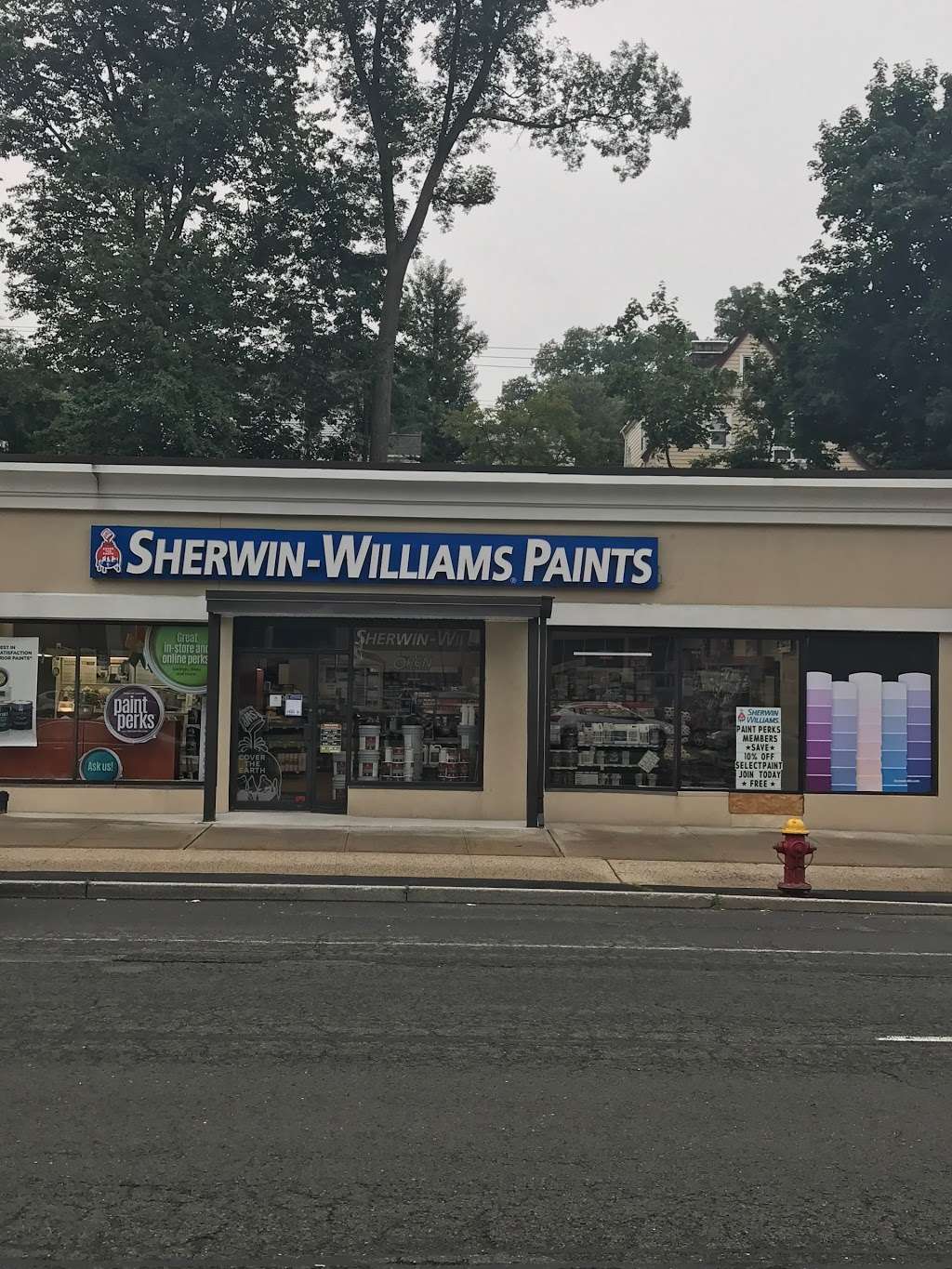The photograph captures the exterior of a Sherwin-Williams paint store. The store is painted beige and is adorned with various advertisements and promotional stickers on its windows, including one that reads "Paint Perks" in blue. The façade features three sets of double-pane windows and doors. The sidewalk in front of the store leads to a four-lane street, or perhaps a parking lot, offering ample space for vehicles. In the foreground to the right of the store’s entrance, a fire hydrant is visible. Beyond the paint store, a cluster of trees forms a natural backdrop, providing a lush green contrast. To the right of these trees, there's a yellow house that peeks through the foliage. The window furthest to the right in the image showcases a selection of paint samples in various shades of purple and blue.